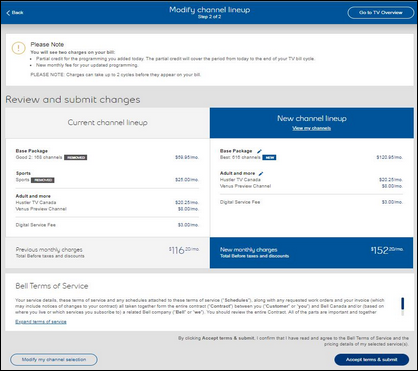The image depicts a screen capture from an online application. The screen has a very pale gray background with various windows in white, accented with blue banners. In the upper left corner, there's a "Back" button with an arrow, set within a blue frame that spans the top of the main window. Centrally within this blue frame, "Modify Channel Lineup" is written in white text.

Beneath this banner, a white horizontal window stretches across the screen, featuring text that begins with "Please note" and continues with smaller, unreadable text. Further down, in bold black text, it says "Review and Submit Changes." Below this section are two adjacent window frames. The left frame has a pale gray background with "Current Channel Lineup" written at the top in black. The right frame features blue horizontal bars at the top and bottom, maintaining a consistent color theme across the interface.